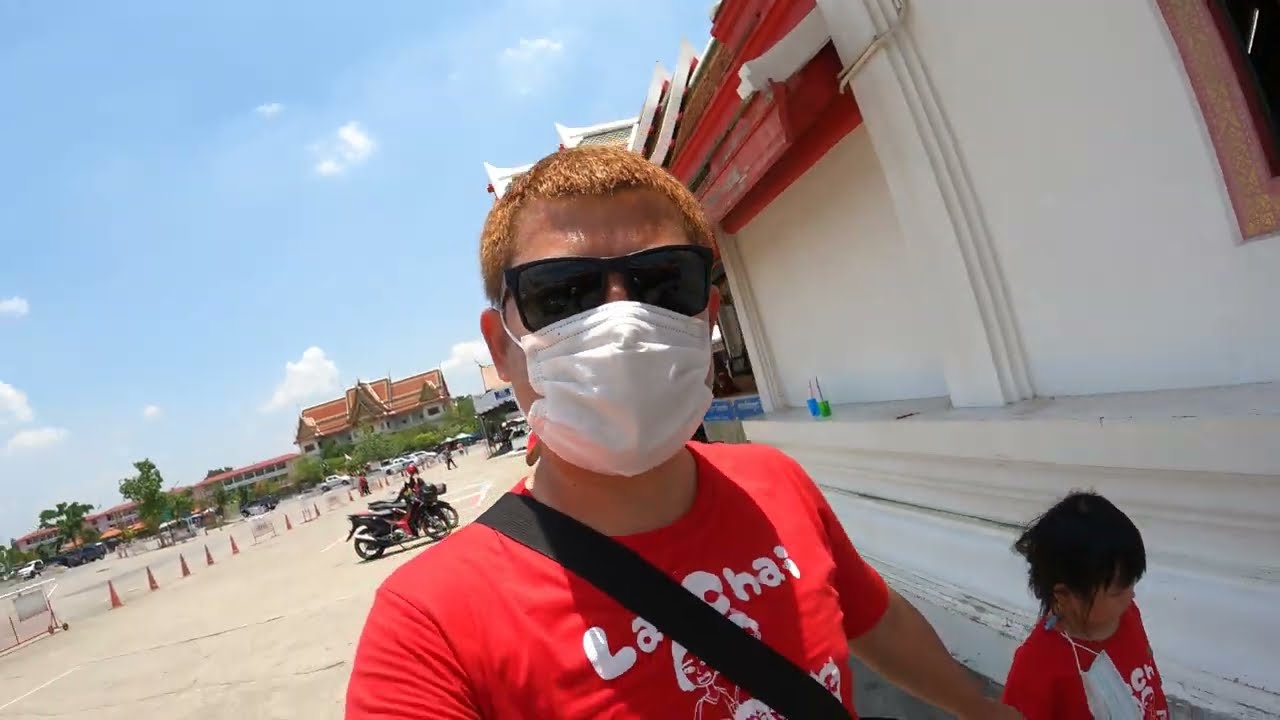In this detailed selfie, a man stands at the center of the image, capturing a moment outdoors in a parking lot. He has extremely short, dyed brown hair and wears black sunglasses along with a white face mask. His red T-shirt, emblazoned with the letters "La Chai" and decorated with cartoon-like family figures, matches that of the small child to his left. This child, who has short black hair and wears a blue face mask hanging down from their face, is also dressed in a smaller-sized red "La Chai" T-shirt. A black strap crosses the man's shoulder, suggesting he might be carrying a case. In the background, two motorcycles are parked near white parking lines, with a series of orange traffic cones and buildings visible in the distance. The scene is brightly lit, indicating it is likely the middle of the day. The setting hints at an outdoor urban environment, possibly an Asian country, with the detailed structures and organized parking lot adding context to the casual yet protected demeanor of the subjects.